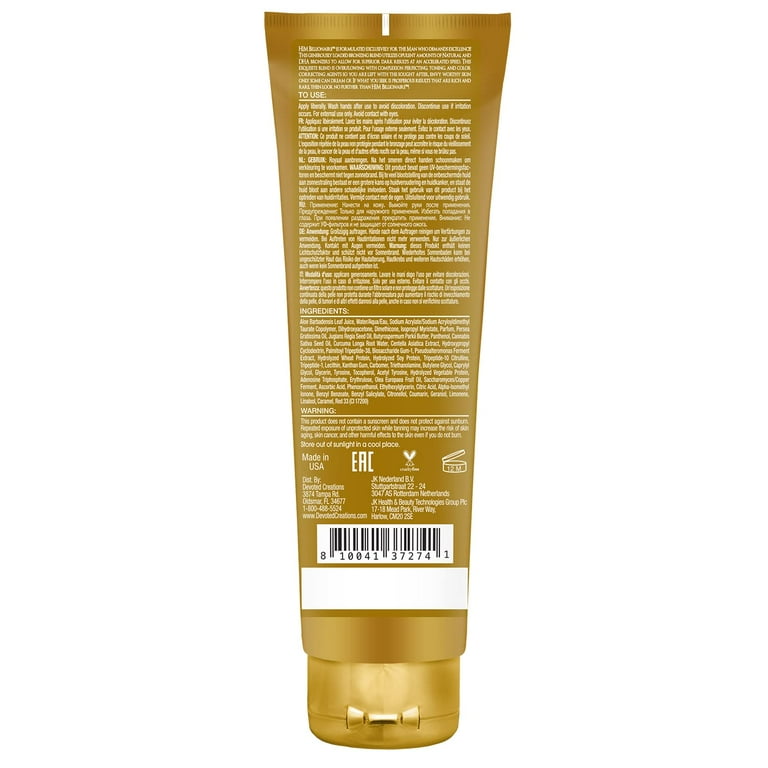The image depicts the backside of a golden tube, likely containing a personal care product such as cream, lotion, or shampoo. This tube features a flip cap at the bottom and is wider at the top where you would squeeze out the product. The tube is covered with extensive, small-text information, including instructions, ingredients, and the statement that it is made in the USA. A prominent "ERC" is displayed towards the bottom. There is also a barcode (UPC: 810041372741) set against a white background, positioned just above a horizontal white stripe running along the bottom of the tube. The entire tube appears golden in color, with white lettering and an additional small vertical white stripe near the top center. The image is well-lit with a clear, white background, highlighting the details sharply.